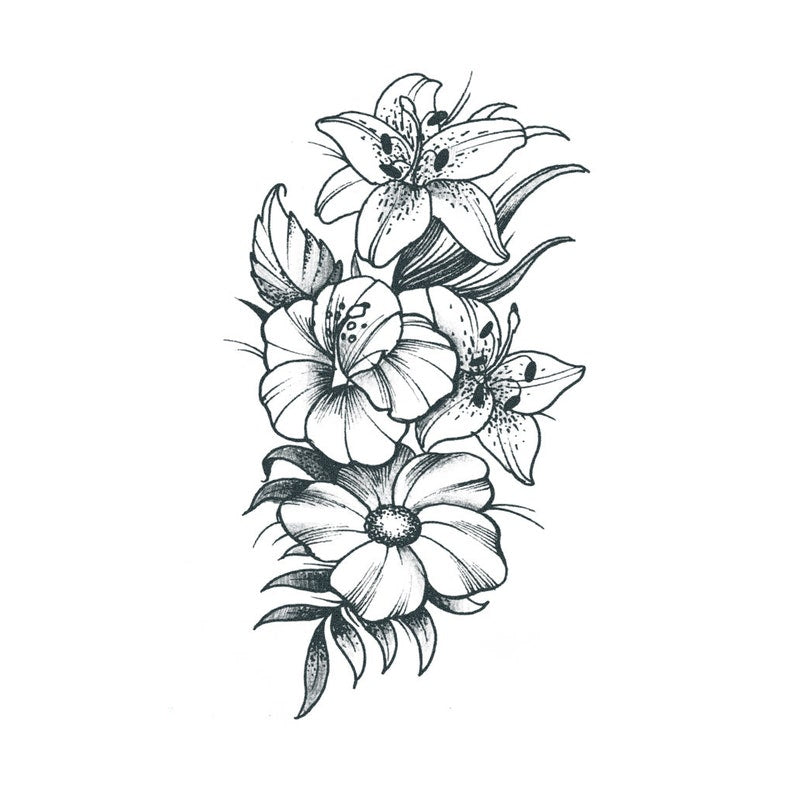The image is a detailed black-and-white pen illustration of four flowers arranged vertically on a plain white background. The flowers vary in type and feature distinct floral structures. At the top, a flower with six petals and three stamens is depicted, accompanied by triangular-shaped leaves. Below it, two flowers are positioned almost side by side. One is characterized by wide, circular petals resembling a sunflower, while the other appears to have the distinctive shape of an orchid with oval pistils and stamen in the center. The bottom flower, also reminiscent of a sunflower, has five thick, pronounced petals surrounding a defined central disk. The illustration displays precise shading achieved through the use of dots and lines, enhancing the texture and detail of the flowers and leaves.